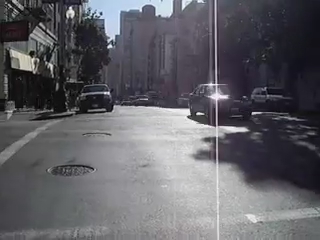This low-resolution photograph captures an outdoor city street scene either at midday or early morning, as suggested by the direction and effect of the sunlight. The scene is taken from the perspective of someone standing in the middle of the street, looking down the road. On both sides of the street, various buildings can be seen, including shopfronts and business facades. Taller buildings, one of which features a steeple or smokestack, are visible in the background. The street itself features two round manhole covers.

Several vehicles are parked on either side of the road, predominantly white trucks and SUVs. In motion on the street is a dark-colored sedan, off which the sun reflects, creating a notable lens flare effect. The sky overhead is clear blue, adding a crisp, bright atmosphere to the image. Additionally, trees with abundant green leaves are visible, with one casting a shadow across the street. The straight white lines of the road markings are clearly visible, adding structure and depth to the scene.